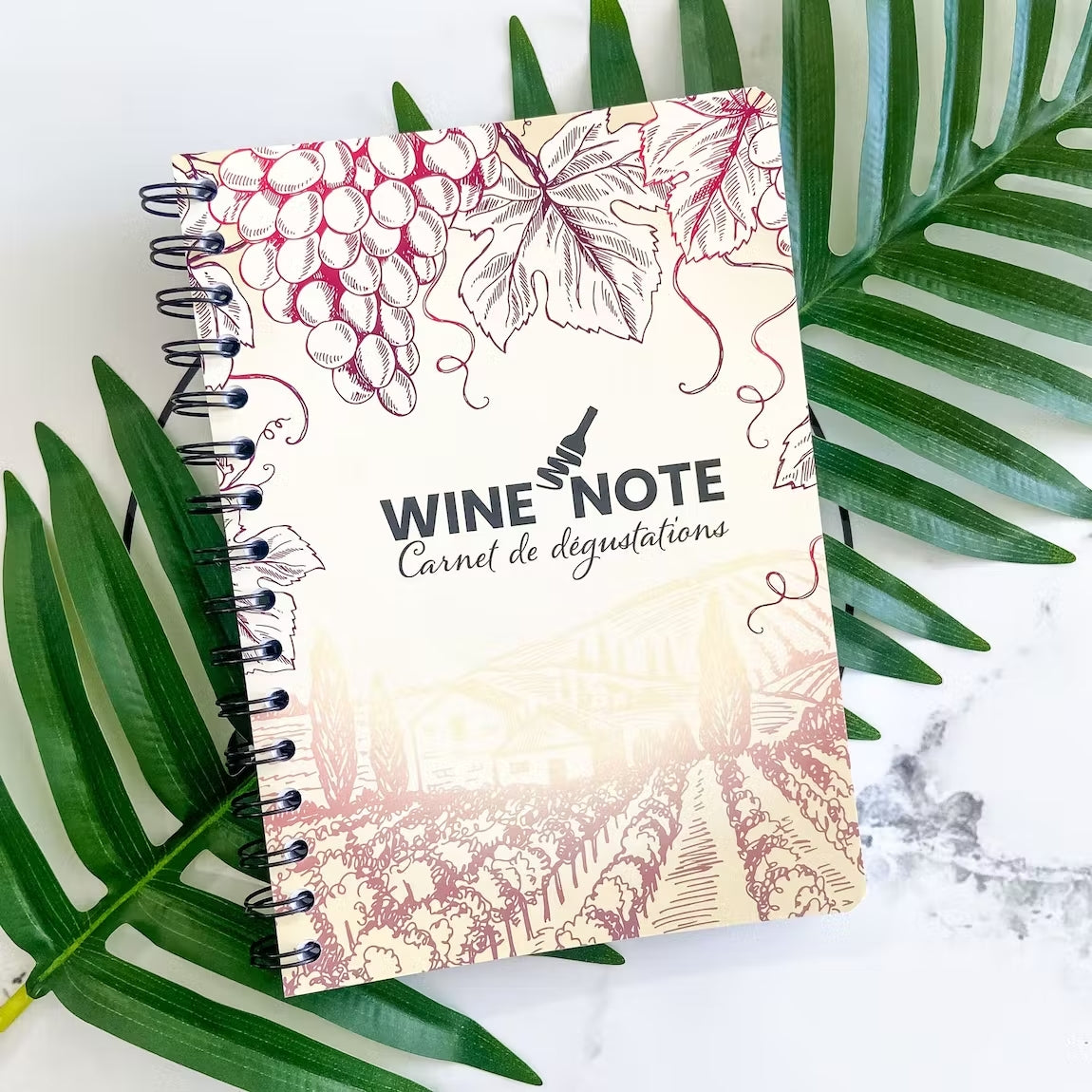This color photograph features a spiral-bound notebook tilted slightly to the left, lying on top of a large green leaf which is placed on a white marble surface. The notebook has a cream-yellow cover adorned with detailed illustrations of grapes, grape leaves, and tendrils. At the bottom of the cover, there is a sketch of a vineyard, complete with buildings, trees, grape vines, and rolling hills. The title on the notebook reads "Wine Note," with a stylized wine bottle, featuring a scribbled label, positioned between the words "Wine" and "Note." Below this title is the phrase "Carnet De Dégustation." The rich maroon and red hues of the cover's illustrations create a striking contrast against the green leaf and the white marble background.